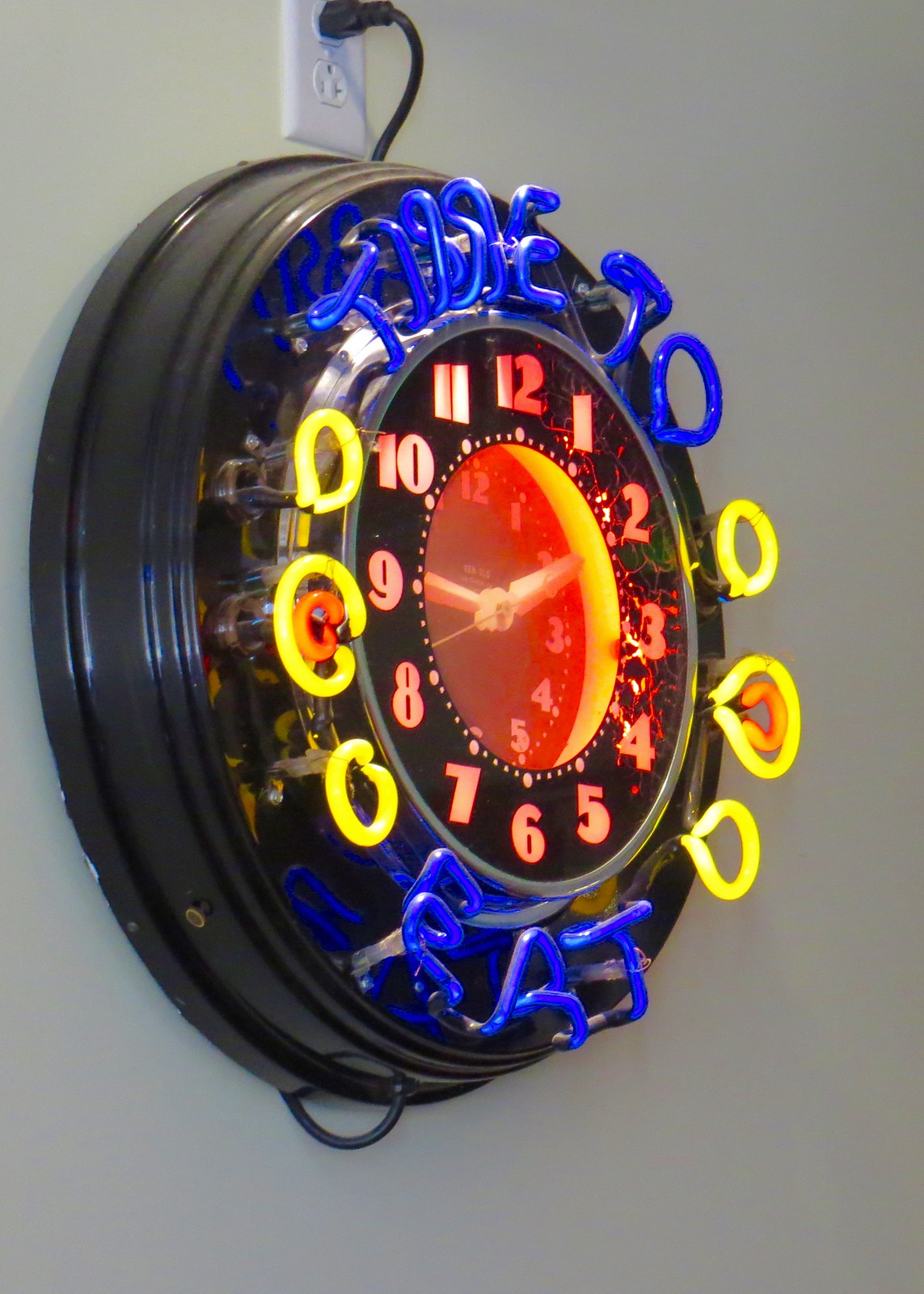This photograph, taken indoors, captures a retro vintage-style analog neon clock mounted on a wall whose creamish-gray coloring is influenced by the lighting. At the top of the image, a white outlet cover is visible with a black cable plugged into it, extending down to power the clock. The clock itself is circular with a black casing and features a prominent neon display. The clock face, which is orange with reddish-orange numbers, is illuminated by vibrant neon lights. 

At the top of the clock, blue neon lights spell out "Time to," and at the bottom, it says "eat," also in blue neon. Surrounding these words are decorative yellow coils of light with hints of orange, forming a visually striking border around the phrase and adding an extra layer of vintage flair. The center of the clock face is a traditional analog clock displaying numbers from one to twelve, with additional smaller circular details enhancing its retro aesthetic.